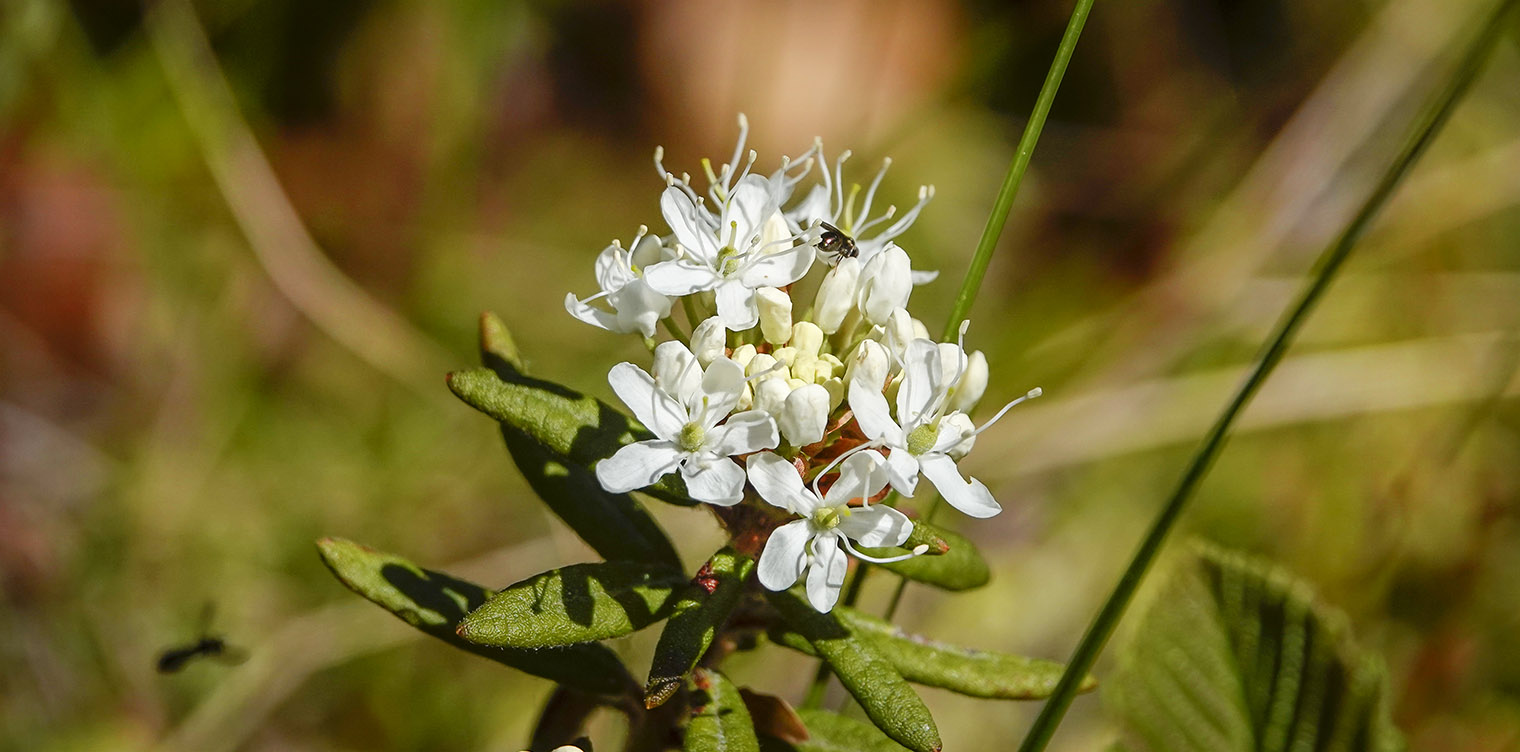The image features a vibrant green succulent plant with some rust-colored and reddish parts. The plant showcases small, white flowers, each with six petals and yellowish-green centers, with thin white stamens extending outward. In one section of the image, a small bee is perched on one of the blooms, adding a touch of life to the scene. The plant's lush leaves, which are pod-like and succulent, are set against a blurred background dominated by hues of green, orange, and tan, hinting at an outdoor environment. In the bottom left corner, the silhouette of another insect is visible, seemingly flying towards or departing from the plant.